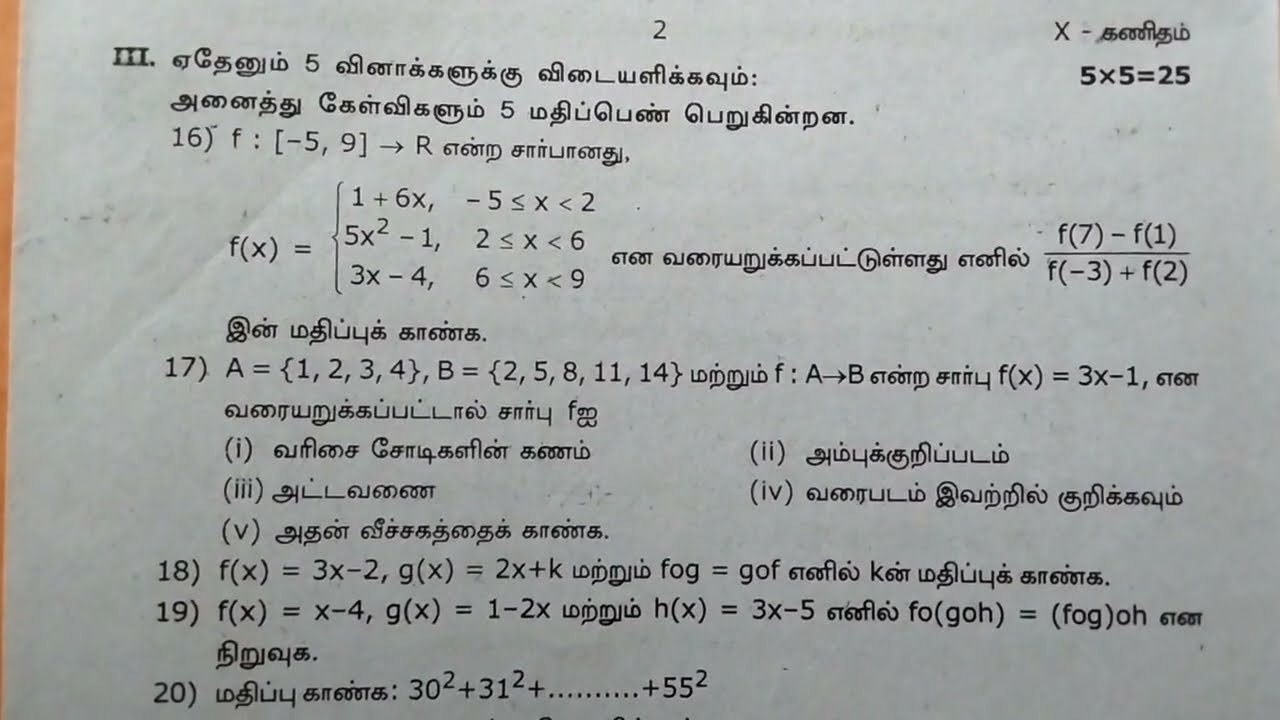This image captures a portion of a math workbook page, featuring complex mathematical equations and explanations. The page is predominantly in a foreign script that resembles Hindi, characterized by its distinctive curves and dots, complemented with Arabic numerals and Roman numerals. At the top left corner, there's a Roman numeral "III," marking the section. Below, the content is organized into five distinct parts labeled 16, 17, 18, 19, and 20. Each section showcases a blend of algebraic equations and written explanations. For example, section 16 includes the expression "16[F: (-5, 9) → R]," followed by more foreign language text. In section 17, the equation "a = [1, 2, 3, 4]" is presented. The equations are neatly handwritten in black ink on white paper, suggesting this might be part of a challenging university-level calculus or algebra exam. Additionally, the upper right corner has a simple arithmetic example, "5 × 5 = 25." The page is labeled "2" at the top center, indicating it's the second page of the document, and some additional text is partially visible at the bottom, hinting at more content beyond what is shown.